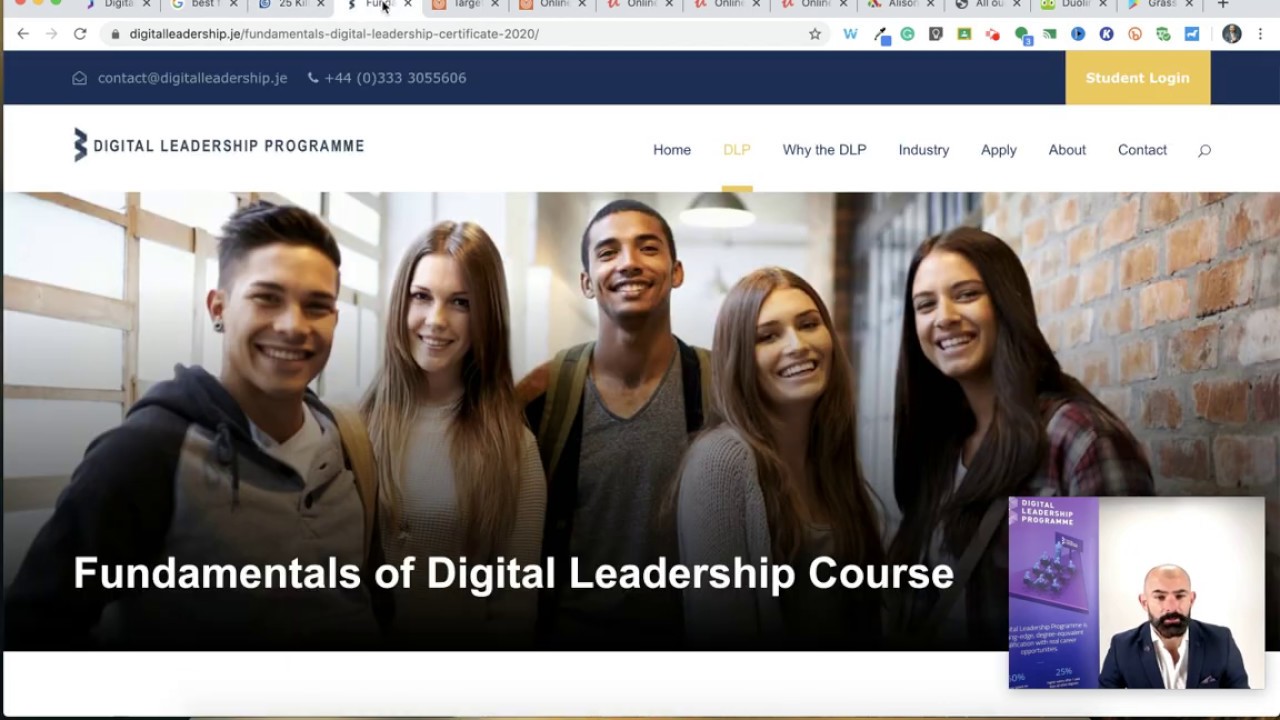The screenshot is from a desktop application displaying a Safari browser window. In the top left corner, the familiar red, orange, and green buttons are visible, allowing users to close, minimize, and maximize the window, respectively. The URL bar prominently displays the web address: "digitalleadership.je/fundamentals/digital-fundamentals-digital-leadership-certificate-2020/". To the right of the URL, there are customized icons for quick access, tailored by the user.

Directly beneath the URL bar, contact information is provided on a navy blue background. The email address, "contact@digitalleadership.je", is displayed followed by a phone number: "+44 (0) 333 3055606", indicating a UK contact.

On the right side, a rectangular light yellow-orange section features a "Student Login" button. Adjacent to this section, on the left, is the text "Digital Leadership Program". Further to the right, a navigation bar includes tabs labeled: Home, DLP (currently selected), Why the DLP, Industry, Apply, About, and Contact. To the far right of the navigation bar, a magnifying glass icon, likely for search, is present.

Below this header section, an image depicts five smiling individuals—two males and three females, likely students—standing in what appears to be a school corridor. The background shows red brick walls, ceiling lamps, and windows, suggesting an indoor walkway.

In the foreground, the title "Fundamentals of Digital Leadership Course" is written in white font, providing a clear indication of the course being highlighted on the webpage.